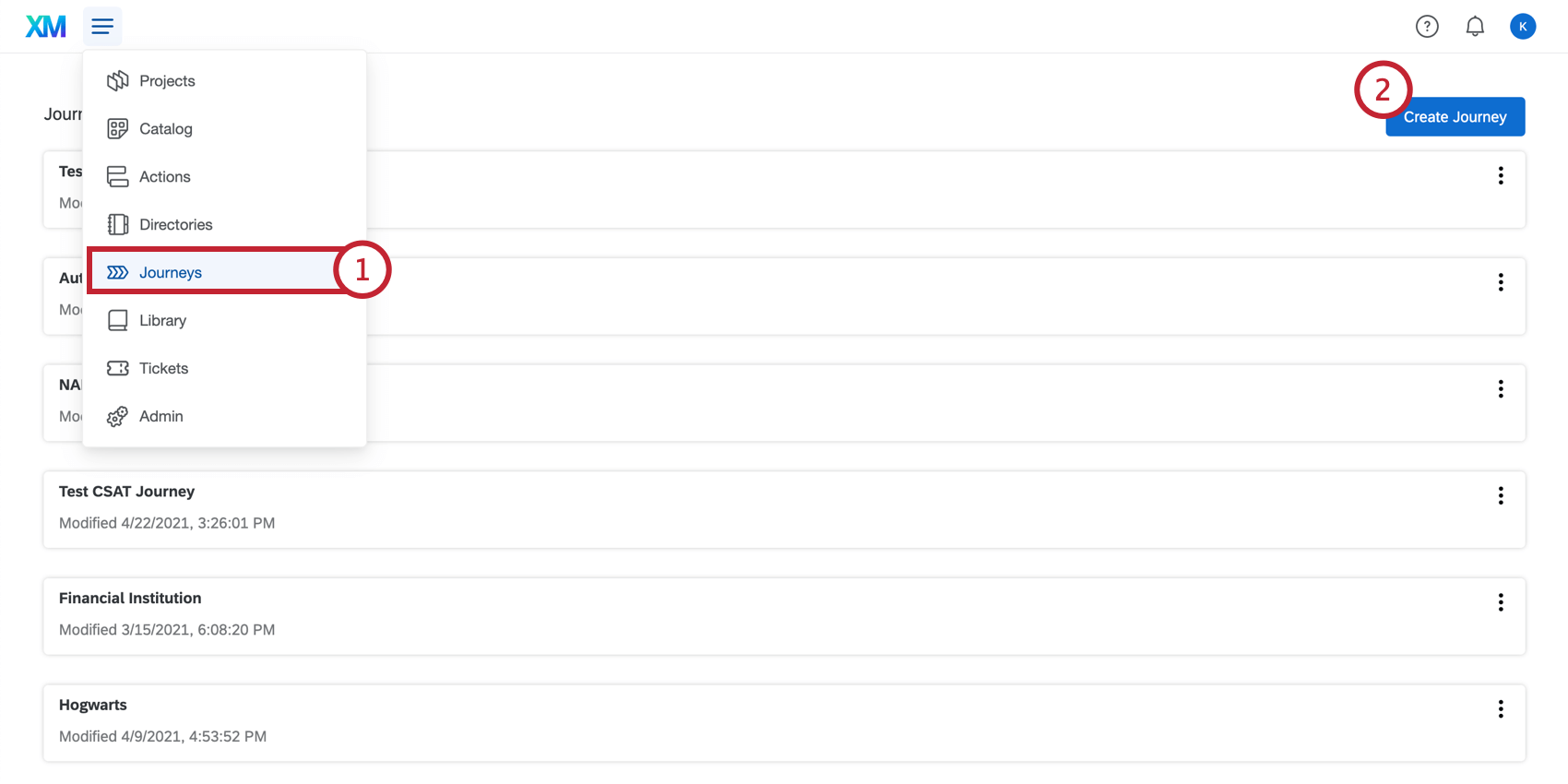This image appears to be a screenshot of a web-based application portal, possibly related to project management or analytics. The layout is wider than it is tall, set against a white background that seamlessly blends into the interface elements akin to Prolific's design. 

In the upper left corner, there is an "XM" logo, beside which a drop-down menu is located. The headings in the menu include "Projects", "Catalog", "Actions", "Directories", "Journeys", "Library Tickets", and "Admin", each accompanied by an icon. The "Journeys" section is highlighted with a red rectangle and a notification circle displaying the number '1'. 

On the upper right side of the interface, a prominent blue button labeled "Create Journey" is also marked with a red circle containing the number '2'. The user is currently logged in, as indicated by the letter "K" in the profile section, which also features a question mark icon (likely for help or support) and a notification bell.

The first three drop-down menu items are partially obscured, making them unreadable. However, the visible menu items include "Test CSAT Journey," "Financial Institution," and "Hogwarts," with each entry displaying modification dates: the "Test CSAT Journey" was last modified on December 20, 2021, at 3:26:01 PM, while "Financial Institution" and "Hogwarts" were modified on March 15, 2021, and April 9, 2021, respectively.

This image seems to provide a snapshot of how users might navigate and interact with various projects or journeys within this specific application. The presence of headings, icons, and modification dates suggests it is designed for efficient project or data management.